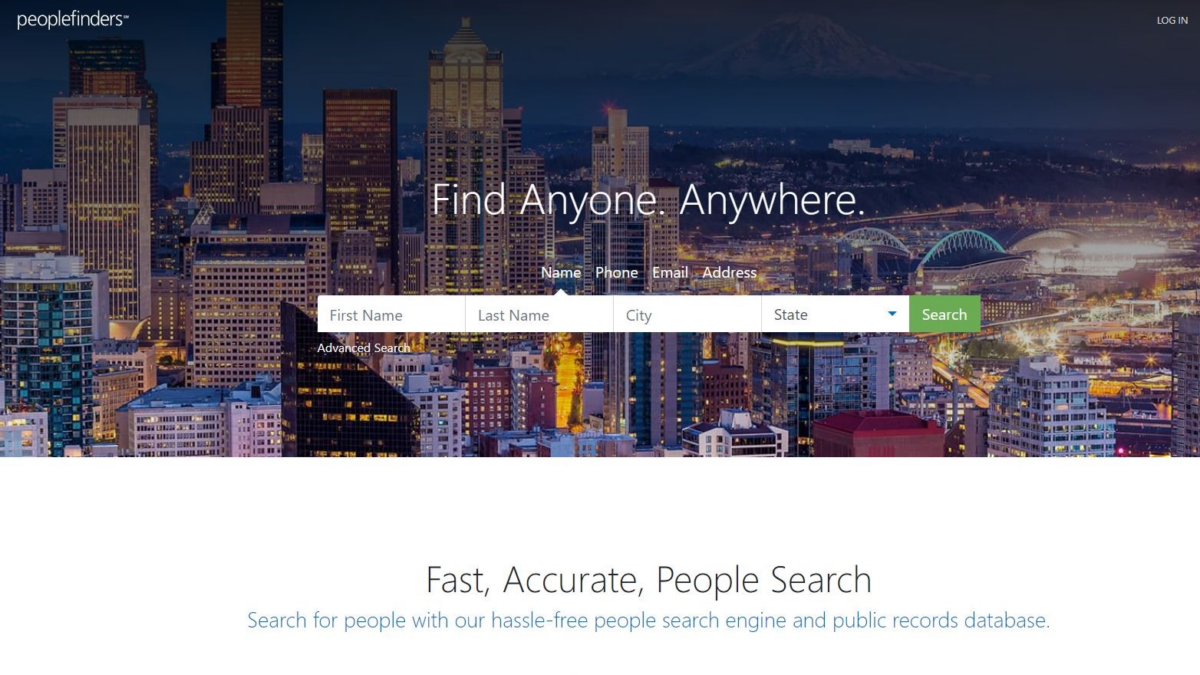This image is a screenshot from the PeopleFinders website. The header features the "PeopleFinders" logo in white text situated on the left, with a "Login" option aligned to the far right. The main section showcases an image of a cityscape at dusk, revealing numerous illuminated skyscrapers and tall buildings with lights glowing in their windows. A distant mountain is visible in the background. 

Overlaying the cityscape, a large white font displays the slogan "Find Anyone Anywhere." Below it, smaller white text describes searchable categories: "Name, Phone, Email, Address." There are text boxes for entering the first name, last name, city, and state, accompanied by a prominent green "Search" button in white font. Further down, an "Advanced Search" option is available in white text.

At the bottom of the image, the phrase "Fast Accurate People Search" is written in large black font, with a smaller blue font beneath it encouraging users to "Search for people with our hassle-free people search engine and public records database."